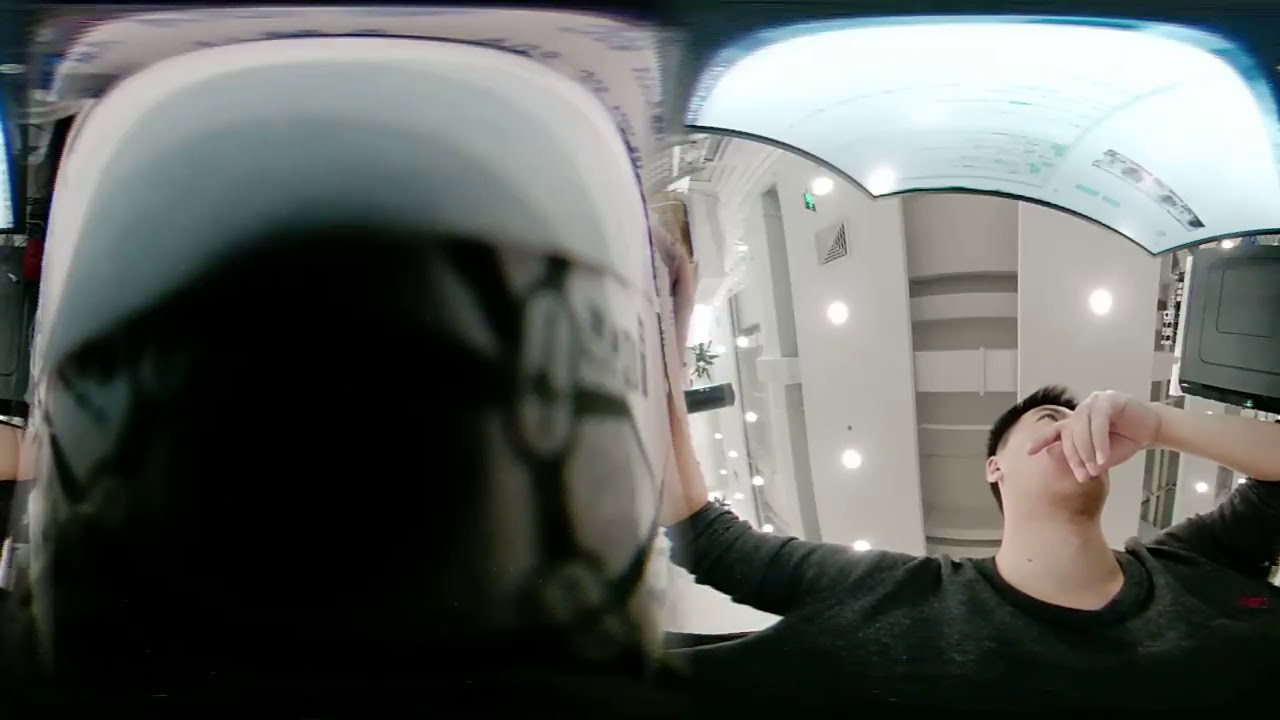In this detailed image, you see a Caucasian man, possibly in his thirties, wearing a dark black long-sleeve shirt with the sleeves pushed up to his elbows. He has dark hair that is pointed near the front. The man is positioned on the right side of the image, and he's holding one arm out, gripping something above his head but away from his body. His left hand is covering his mouth, giving a sense of contemplation or concern, and his head is tilted back slightly as he looks up and to the right. He is intently focused on a screen that displays some digital items, which are not readable due to the image being potentially upside down. The setting is a small room with a light gray ceiling, featuring circular lights and ventilation. On the left side of the image, there is an unclear, possibly distorted, object that resembles a light blue and black or white mask or container with rounded corners. The image appears to be taken from a low angle, giving a sense of looking upward at the scene.